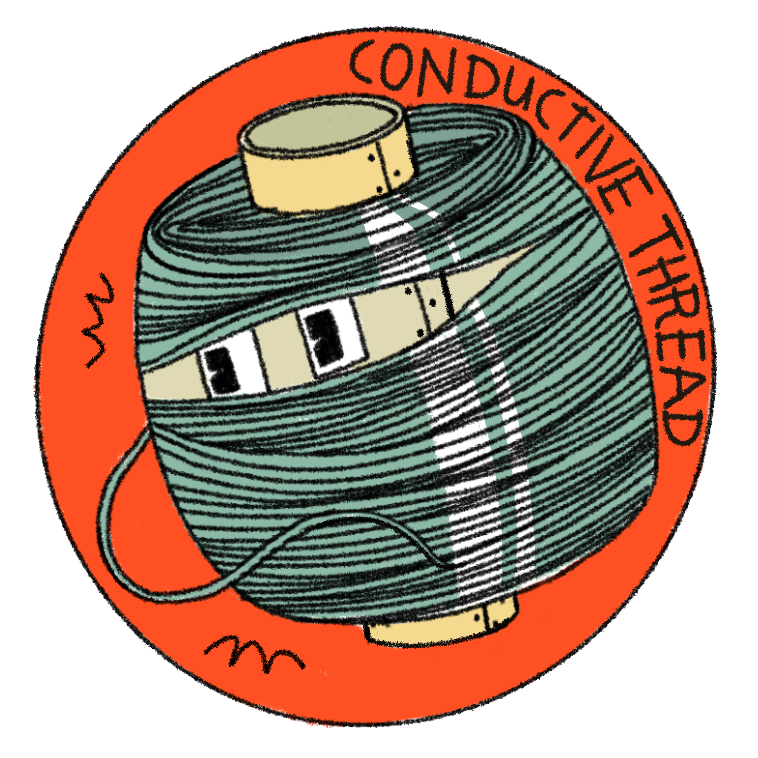This image features a vibrant, digitally-created design centered on an orange circle outlined in black. On the right-hand side, black text reads "conductive thread." At the heart of the image is an animated figure resembling a little robot or creature, comprised of a green cylindrical form with yellow stripes. This form is outlined in black thread, and its 'head' is slightly open, revealing two square, white eyes with black pupils staring sideways. Above the eyes, a cone-like structure with three dots and one line protrudes, while a similar cone at the bottom shows just two dots and one line slightly visible. Surrounding this central figure, there are several squiggly, black lines on the left. The overall artistic impression is whimsical, blending text and visual elements to depict the dynamic concept of conductive thread, complete with a sense of motion and character.